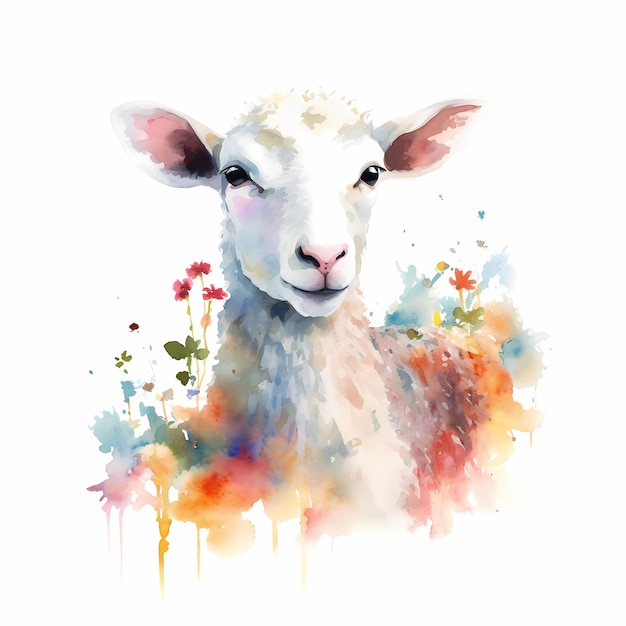This image is a detailed watercolor painting of a sheep, set against a stark white background. The sheep, portrayed from the chest upwards, is predominantly white with subtle beige spots on the top of its head. The inner portions of its ears and its nose are a delicate pink. The sheep's head is slightly tilted as it gazes off to the right. Beginning from its belly, the artist has whimsically incorporated an array of colors into the sheep's body, mainly featuring shades of light brown, mauve, oranges, reds, and blues. This creative use of color creates a gradient effect that extends outward, transitioning into scattered blobs. Surrounding the sheep are various flowers, predominantly pink, with a singular orange flower and some red, pink, and yellow flowers, accented by green leaves, adding a touch of natural beauty to the scene.